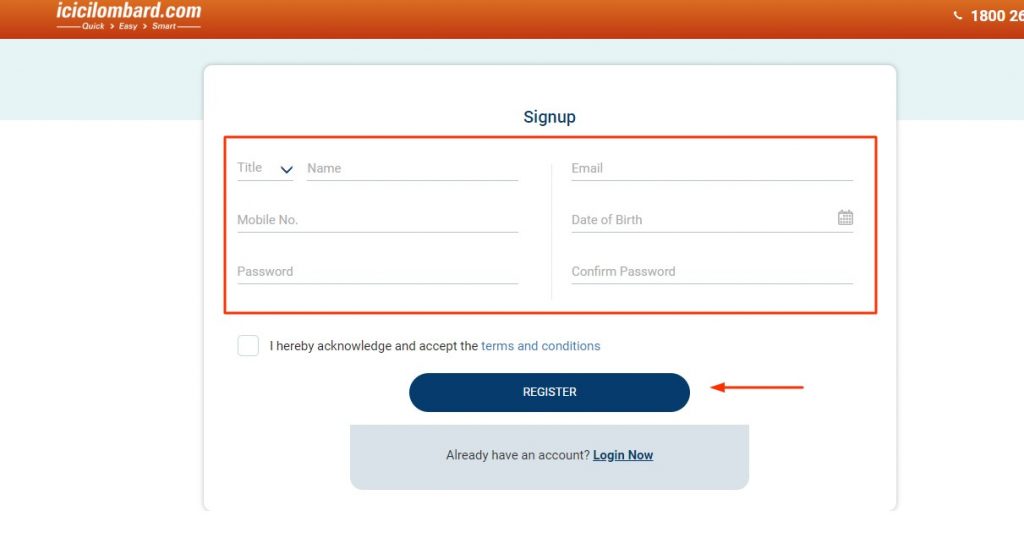The image is a screenshot of a website signup page from ICCLombard.com. Featured prominently in the upper left corner, the website's name, "ICCLombard.com," is displayed in white font against an orange background. Directly beneath it, the tagline "Quick, Easy, Smart" is written in the same font and color scheme. In the upper right corner, similarly styled with white text on an orange background, is the start of the business's phone number, "1-800-26," though the rest of the number is cut off by the edge of the image.

At the center of the image is a white dialog box where users can sign up for the website. The top of the signup box features the heading "Sign Up" in dark blue text. Directly below this header is a dark orange rectangular box matching the shade of the orange from the header bar hosting the website's name. The signup box includes input fields for the following information: Title, Name, Email, Mobile Number, Date of Birth, Password, and Confirm Password.

Additionally, there is a checkbox for users to acknowledge and accept the terms and conditions. Completing the signup form is a navy blue call-to-action button labeled "Register" in white text. The overall layout is user-friendly and visually cohesive, emphasizing ease of use and clarity.